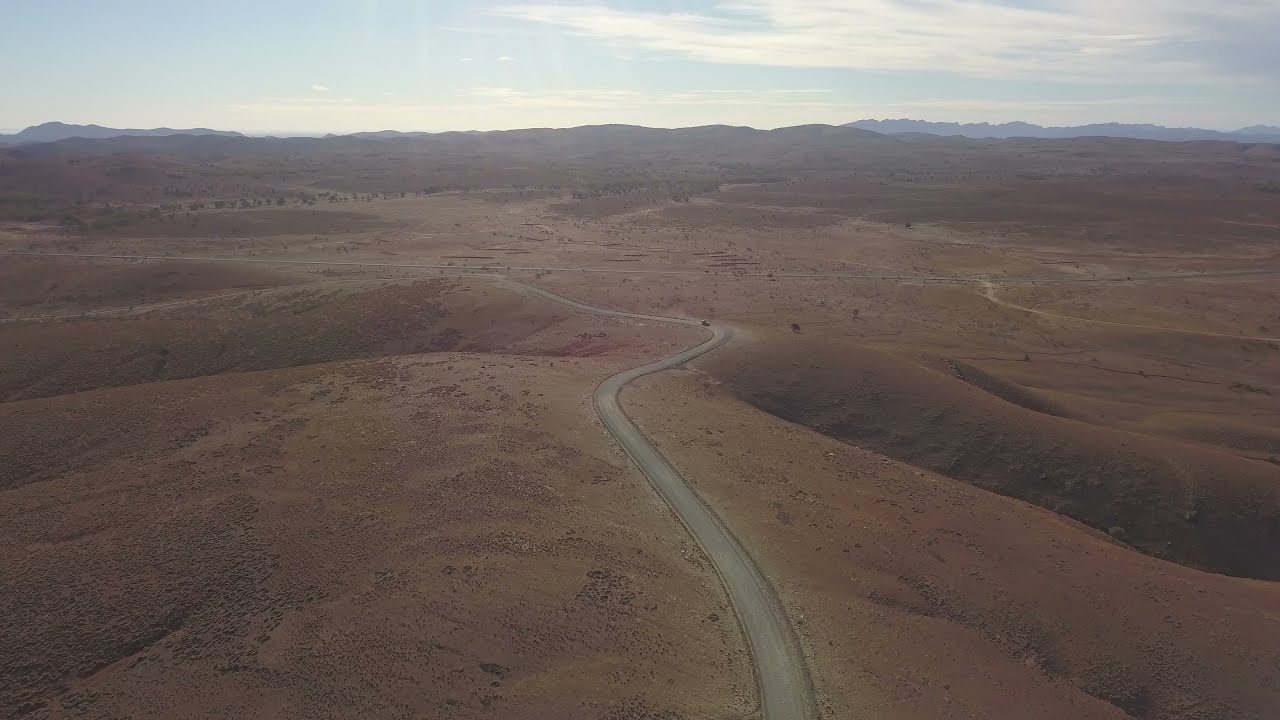The image captures an overhead view of a vast, brown desert landscape on a partly cloudy, hazy day. The rugged terrain features hills, valleys, and large crevasses that give a wavy appearance to the sandy, dirt-covered ground. Running through the center of the image is a single, curvy, gray paved road that stretches towards the horizon in the upper fourth of the frame. The lower right corner of the image displays a shadow that creates the illusion of a crevasse in the landscape. The sky above is blue with scattered white clouds, and while the sun itself is not visible, rays and flares are evident towards the top middle of the image. In the distance, faint mountains can be seen through the haze, with no signs of human or animal presence, adding to the vast, untouched feel of the scene.